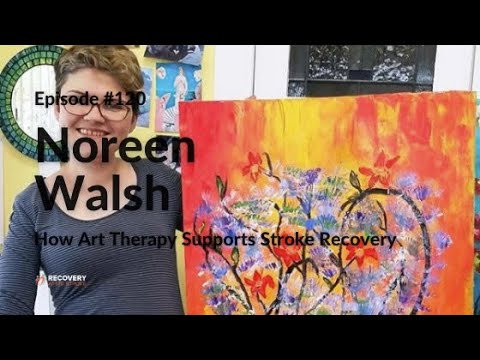This image is a title card for episode 120 featuring Noreen Walsh titled "How Art Therapy Supports Stroke Recovery." The main focus of the image is a smiling woman with short brown hair and glasses, wearing a dark, thin-striped shirt. She is holding up a large, colorful painting. The background of the painting is vividly decorated with thick brush strokes of orange, red, and yellow. Central to the painting is an arrangement of red, purple, and yellow flowers with green leaves and black stems, artistically forming a heart shape on one side. Behind her, there is a yellow wall adorned with various pictures and a distinctive green circle. The episode title is prominently displayed across the image in black font, which can be slightly challenging to read against the vibrant background.